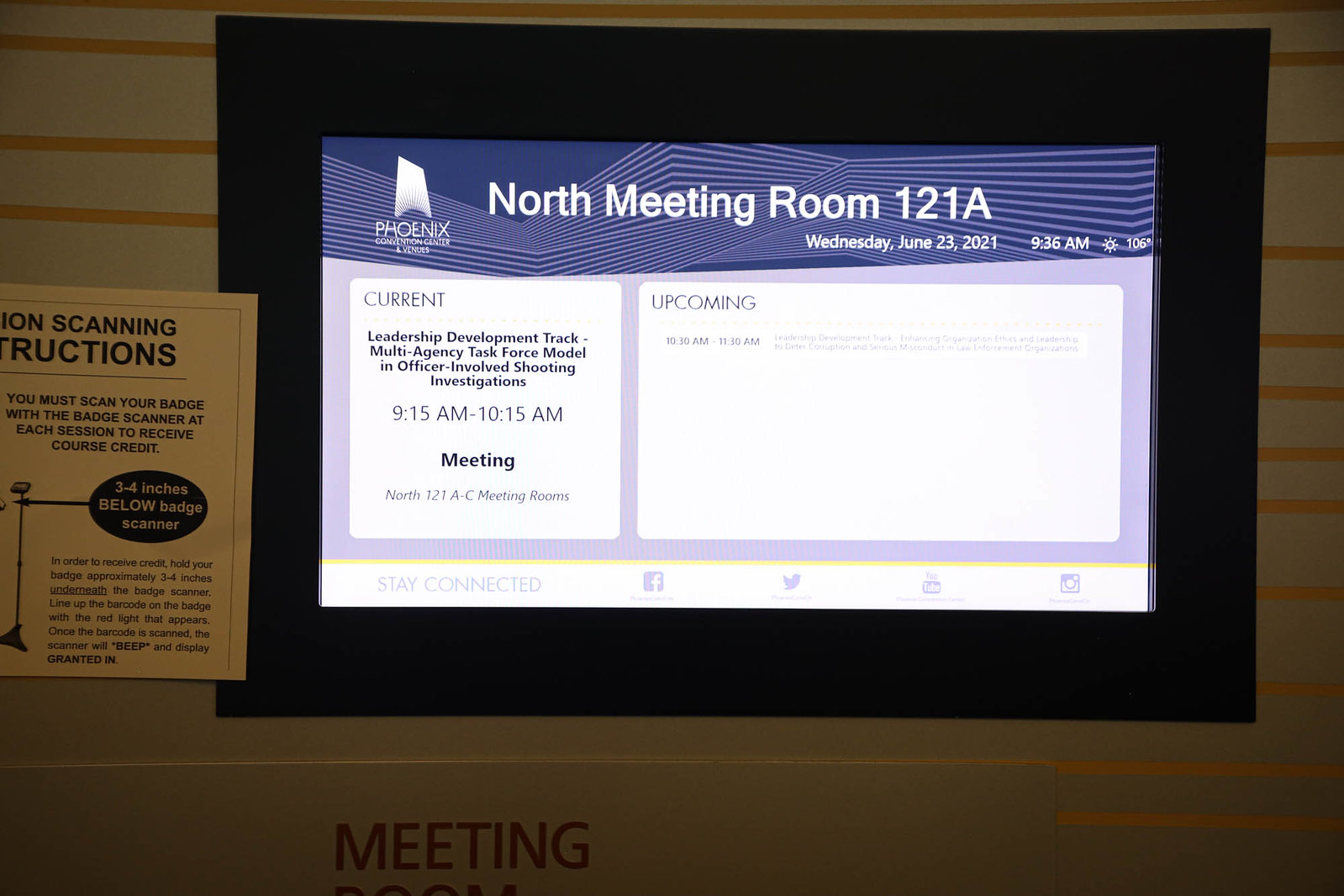The image captures a projector screen displaying detailed event information at the Phoenix Convention Center, specifically in the North Meeting Room 121-A. The top left of the screen reads "Phoenix Convention Center" with text beneath stating the location as "North Meeting Room 121-A." The date and time are noted as "Wednesday, June 23, 2021, 9:36 a.m." along with the temperature, "106 degrees," accompanied by an image of the sun.

Beneath this information, the screen is divided into two sections. The left section, titled "Current," details a scheduled session: "Leadership Development Track: Multi-Agency Task Force Model in Officer-Involved Shooting Investigations" from "9:15 a.m. to 10:15 a.m." in "Meeting North 121-A-C Meeting Rooms." 

The right section, labeled "Upcoming," lists a future event at the conference, though the text is too small to be legible. Additionally, nearby is a piece of paper with scanning instructions, reminding participants to "scan your badge with the badge scanner at each session to receive course credit."